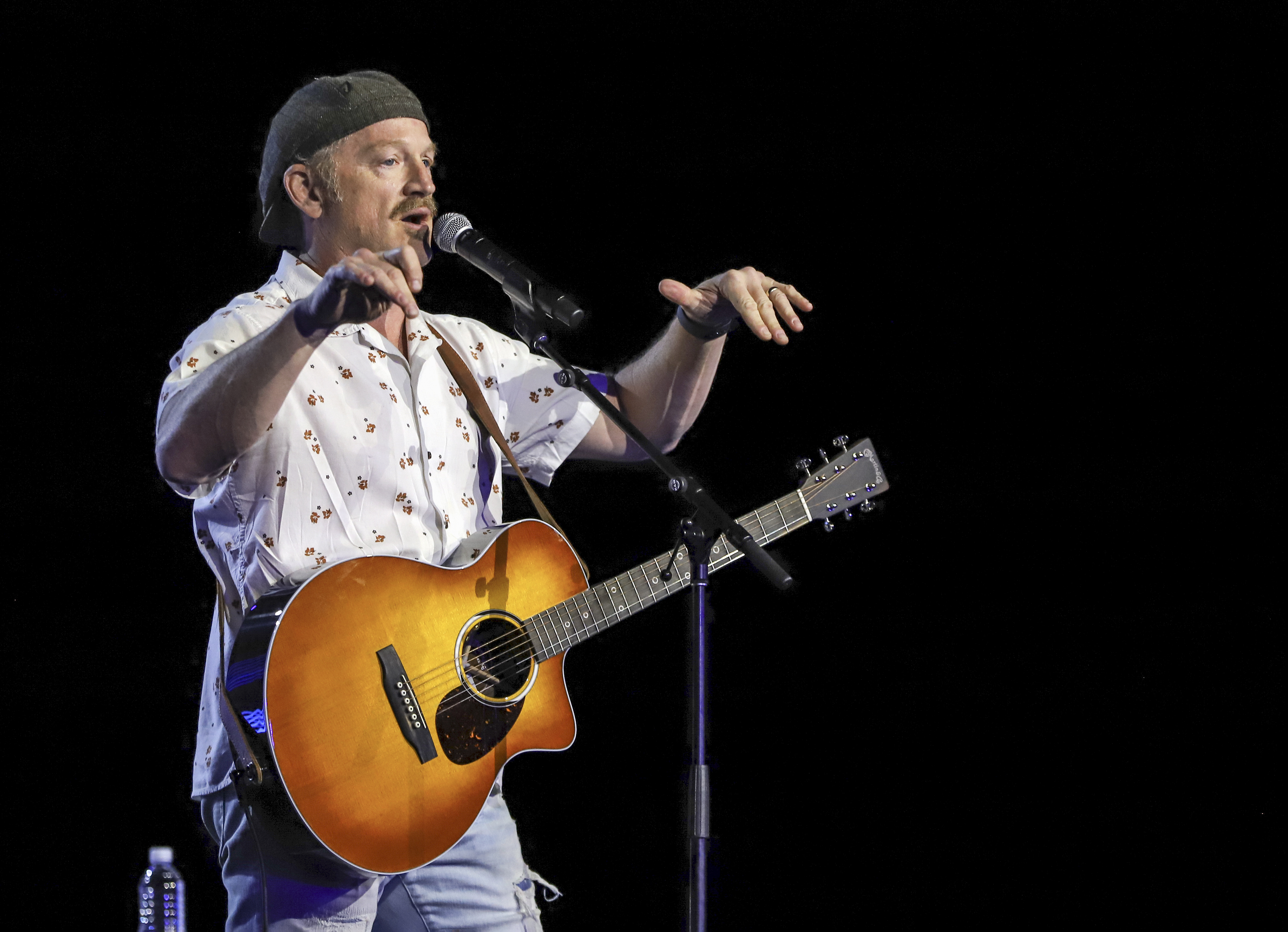In the photograph, an older white man stands on stage, his presence captured in a moment of what appears to be a musical performance or a speech. His attire consists of a white button-up shirt adorned with orange flower patterns, short sleeves, and a turned-down collar. Complementing his shirt, he wears blue jeans that feature multiple tears on the front. On his head, he has a gray cap with the bill facing backwards. The background is pitch black, giving the illusion that he is standing in a void. Positioned to the left of his leg is a clear plastic water bottle with a white cap. In front of him is a purple microphone stand with a black upper arm, ending in a silver-headed black microphone. A brown guitar strap rests on his shoulder, holding a brown acoustic guitar. Both of his hands are raised at shoulder height, open and possibly gesturing to the audience, and he is wearing a ring on his left ring finger. The subdued lighting focuses all attention on the man and his actions, drawing viewers into the scene.